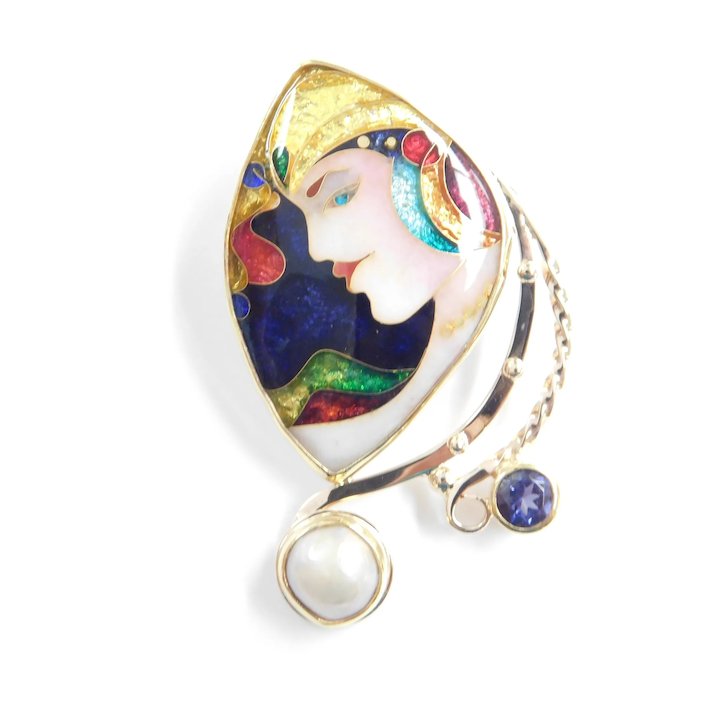This detailed brooch features a central design of a woman's face with blue eyes and lips, adorned with what appears to be a gold cap or hair. Her portrait is set against a navy blue background, surrounded by intricate patterns of gold, red, and green colors. Extending from the main part of the brooch is a gold chain that holds a secondary gold piece, which is embedded with tiny stones and ends with a dangling element featuring a pearl. The brooch, primarily golden in color, also showcases a range of hues including turquoise, beige, pinkish tones, and white, reflecting an elaborate and colorful piece of jewelry that could have either a vintage or contemporary origin.